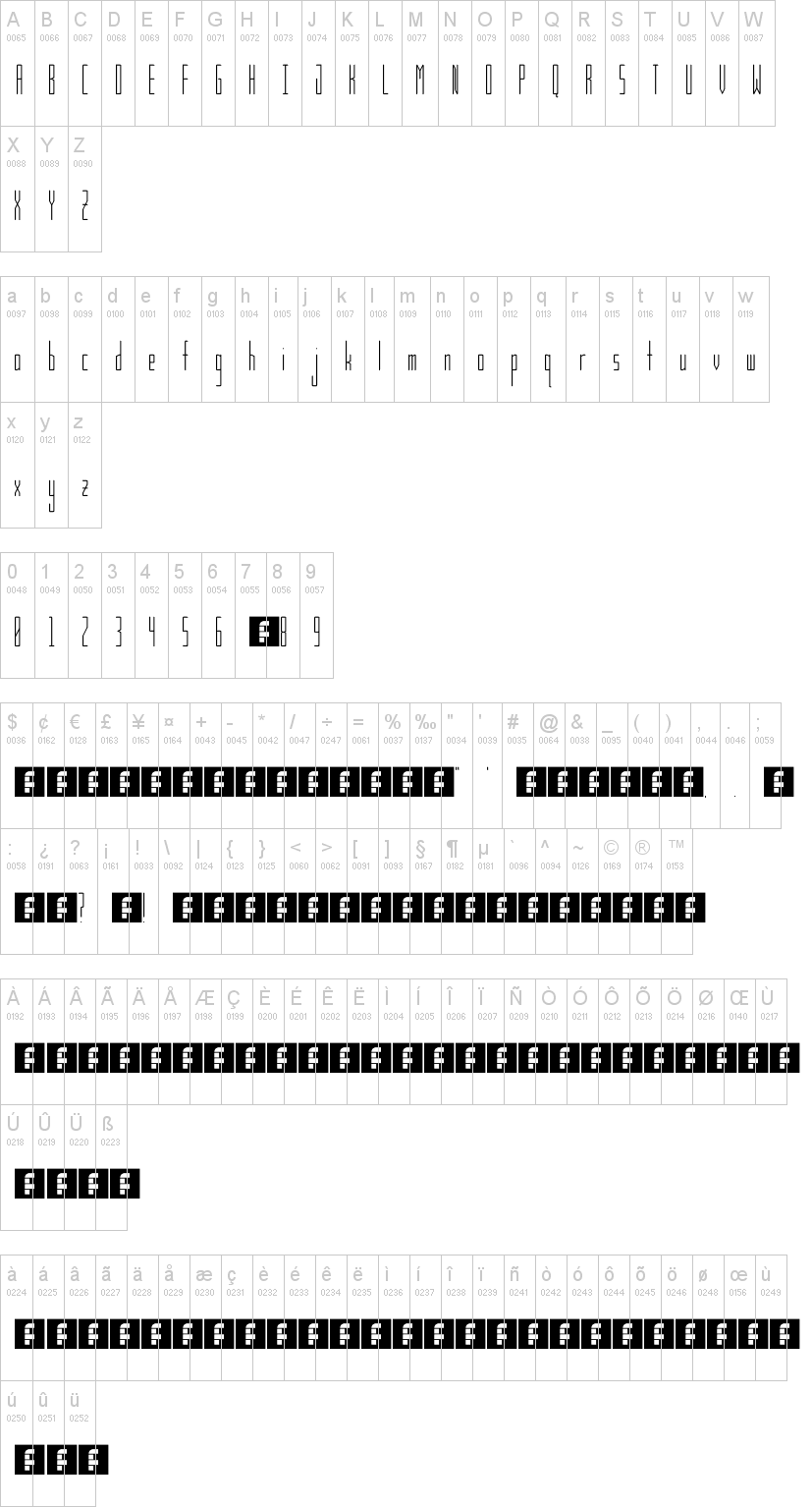The image depicts an extensive array of vertically oriented rectangles arranged in orderly rows that seemingly extend into the horizon. Each rectangle is uniformly divided into two segments: the top section features a lighter gray background with a unique alphanumeric code starting with "A0065" and appearing consistently on each rectangle. The code is inscribed in a light color, denoting a sequence. Below this, stark black letters and corresponding numbers sequentially progress from "A" with "B0066", followed by "B" with "C0067", continuing alphabetically. These black markings differentiate each rectangle, marking the progression with "C", "D", "E", so forth until "L0076".

Towards the bottom of the arrangement, the configuration alters slightly, presenting a new sequence beginning from "A0097" to "B0098", while still adhering to the same format of a gray alphanumeric code atop and black letters underneath. This systematic display repeats uniformly, creating a methodical and vast visual alignment of labeled rectangles.